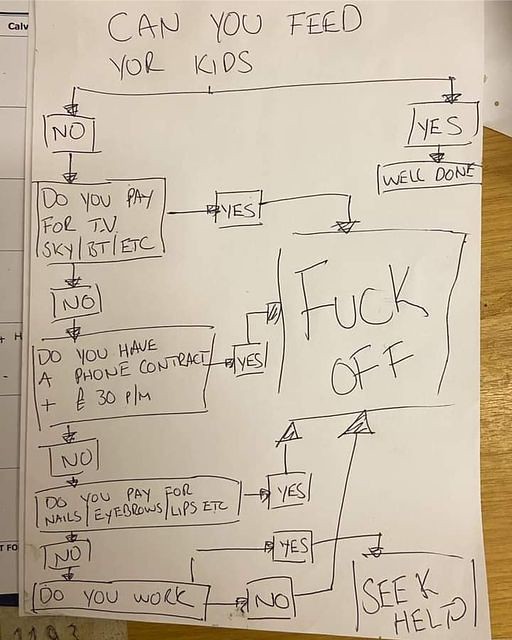The image depicts a handwritten flowchart on a piece of printer paper, created with black ink, and photographed from above on a wooden table. The chart outlines a decision-making process regarding the misappropriation of money, particularly focusing on whether individuals can feed their children. 

The top of the flowchart begins with the question "CAN YOU FEED YOUR KIDS?" in capital letters. If the answer is "YES," an arrow leads to a box that says "WELL DONE." If the answer is "NO," the chart asks, "DO YOU PAY FOR TV, SKY, BT, ETC.?" If the answer here is "YES," it directs to a box labeled "FUCK OFF." If "NO," it proceeds with, "DO YOU HAVE A PHONE CONTRACT PLUS £30 P/M?" A "YES" answer again leads to the "FUCK OFF" box, while "NO" prompts the question, "DO YOU PAY FOR NAILS/ EYEBROWS/ LIPS, ETC.?" A "YES" answer leads to the same dismissive "FUCK OFF" box. If the answer is "NO," the final question asks, "DO YOU WORK?" If the response is "NO," it also directs to the "FUCK OFF" box. If the answer is "YES," it concludes with a box that says "SEEK HELP."

The flowchart uses minimal color, primarily white and gray, with the written text in black.